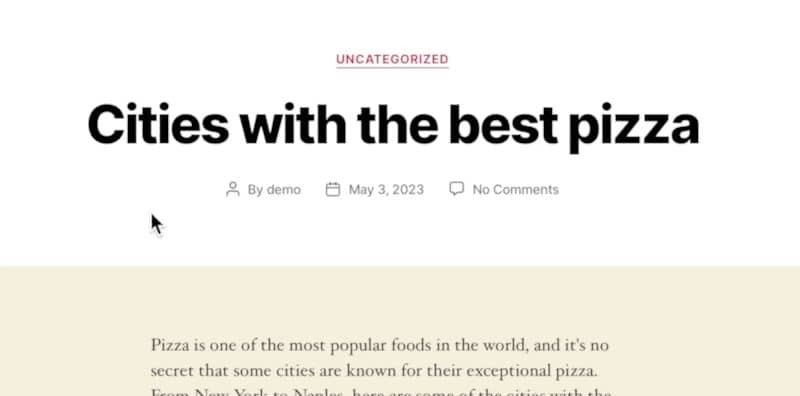The image is a screenshot showcasing the top segment of an article. The header prominently labels the article under "Uncategorized". The article title reads, "Cities with the Best Pizza by Demo Made, 2023," and it notes that there are currently no comments. Below the title, a brief excerpt from the article is visible, set against a pale yellow background. The text begins, "Pizza is one of the most popular foods in the world and it's no secret that some cities are known for their exceptional pizza," before being cut off, suggesting a detailed exploration of global cities celebrated for their outstanding pizza offerings.